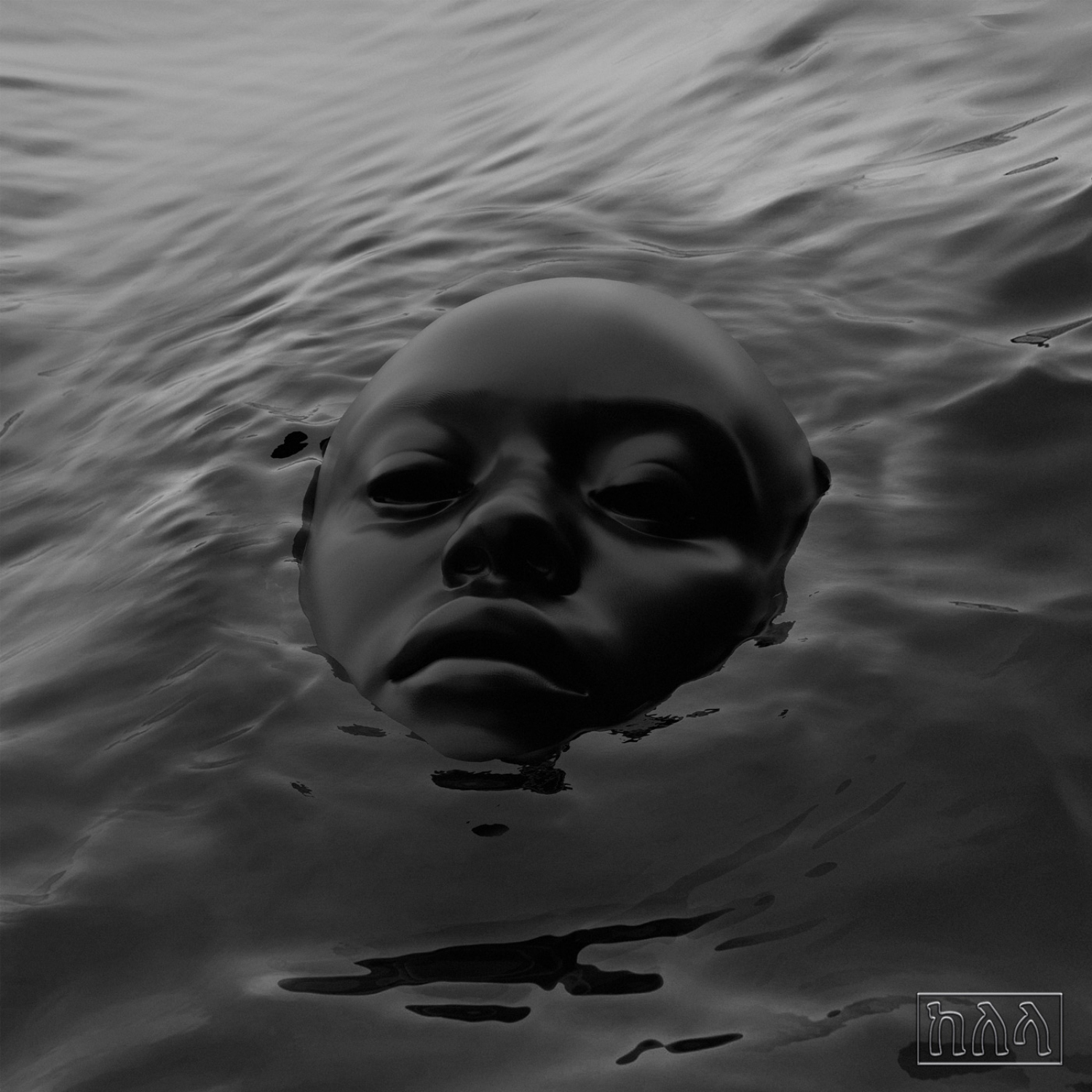The image is a stylized, black-and-white 3D rendering of a face emerging from or submerging into a thick, black liquid. The face, which is androgynous and devoid of any distinguishable features like eyes or hair, appears highly polished and reflective. Only the area from the chin to just above the forehead is visible, enhancing the surreal quality of the artwork. The black liquid surrounding the face has subtle ripples, adding a touch of realism to the scene. In the bottom right corner, there are three unusual symbols; two resemble horseshoes, while the one on the left looks like an 'N' with an additional stroke. The overall composition is dark and enigmatic, with lighter reflective highlights on the top left of the water.